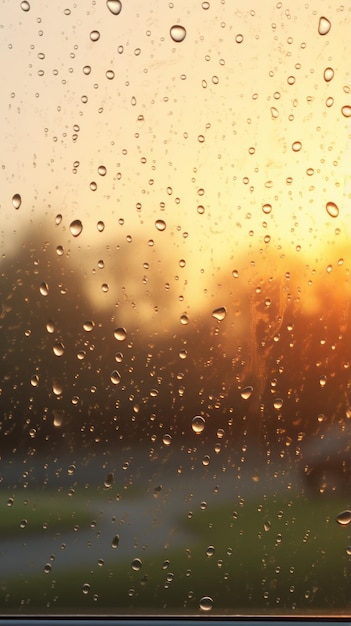The image captures a close-up view of a rain-streaked window pane, covered in hundreds of raindrops varying in size. Through the blurred glass, you can make out a driveway leading to a green lawn and tall trees in the background. To the right, part of a vehicle is faintly visible. The scene outside appears to be during a sunset, transitioning from a bright pink sky at the top to a darker yellowish-orange near the horizon, adding a warm glow to the surroundings. The picture seems to have been taken from the inside, possibly from within a vehicle or a house, suggesting a serene, rain-soaked evening.